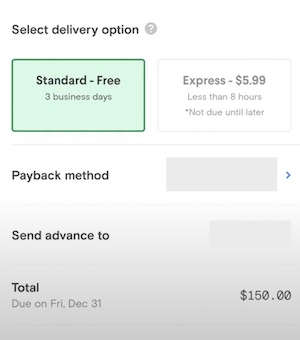This image captures the screen of a cell phone displaying a page where the user is selecting a delivery option. At the top of the screen, "Select Delivery Option" is prominently displayed in black text, accompanied by a gray circle with a white question mark icon to the right. Below this header, on the left side, the screen presents a green box labeled "Standard - Free" in black text, with "3 business days" noted in gray text beneath it. 

To the right of this option, there is a white box labeled "Express - $5.99" in black text, with "less than 8 hours" written in gray text beneath it. Additionally, there is a small star indicating that this option is not due until later. The user has selected the "Standard - Free" option.

Further down the page, there is a section titled "Payment Method" with a gray rectangle next to it, featuring a small blue arrow pointing to the right. Below this, another line reads "Send advance to," followed by a clickable gray rectangle. At the bottom of the screen, the total amount due is displayed, stating "Due on Friday, December 31st" with the amount "$150."